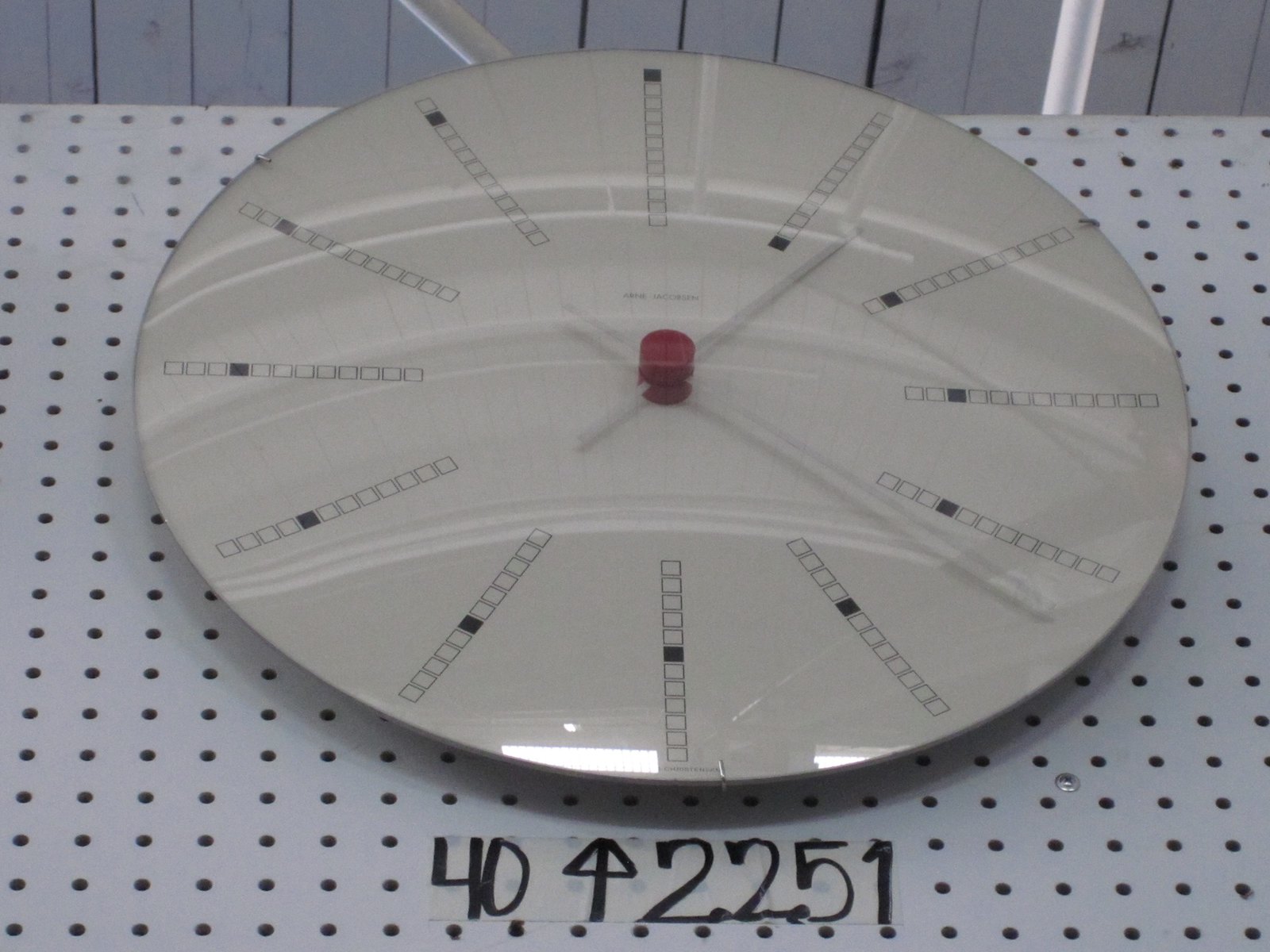This color photograph features a medium-sized, stylized circular clock mounted on a white pegboard wall that has numerous small holes throughout it. The clock has a clear glass cover and a striking design, with no traditional numbers. Instead, twelve lines of white squares represent the hours, each having one black square filled in to indicate the current hour. In the clock’s center is a small red circle from which the slim, white hands of the clock extend, currently pointing to approximately 1:23. Visible at the top of the image, part of the ceiling appears to be white wood. Below the clock, attached to the pegboard, is a piece of tape with black writing. The tape displays the number "40" with a black arrow pointing upwards next to it, and the number "2251" to the right of the tape. The photo does not include any people or animals.